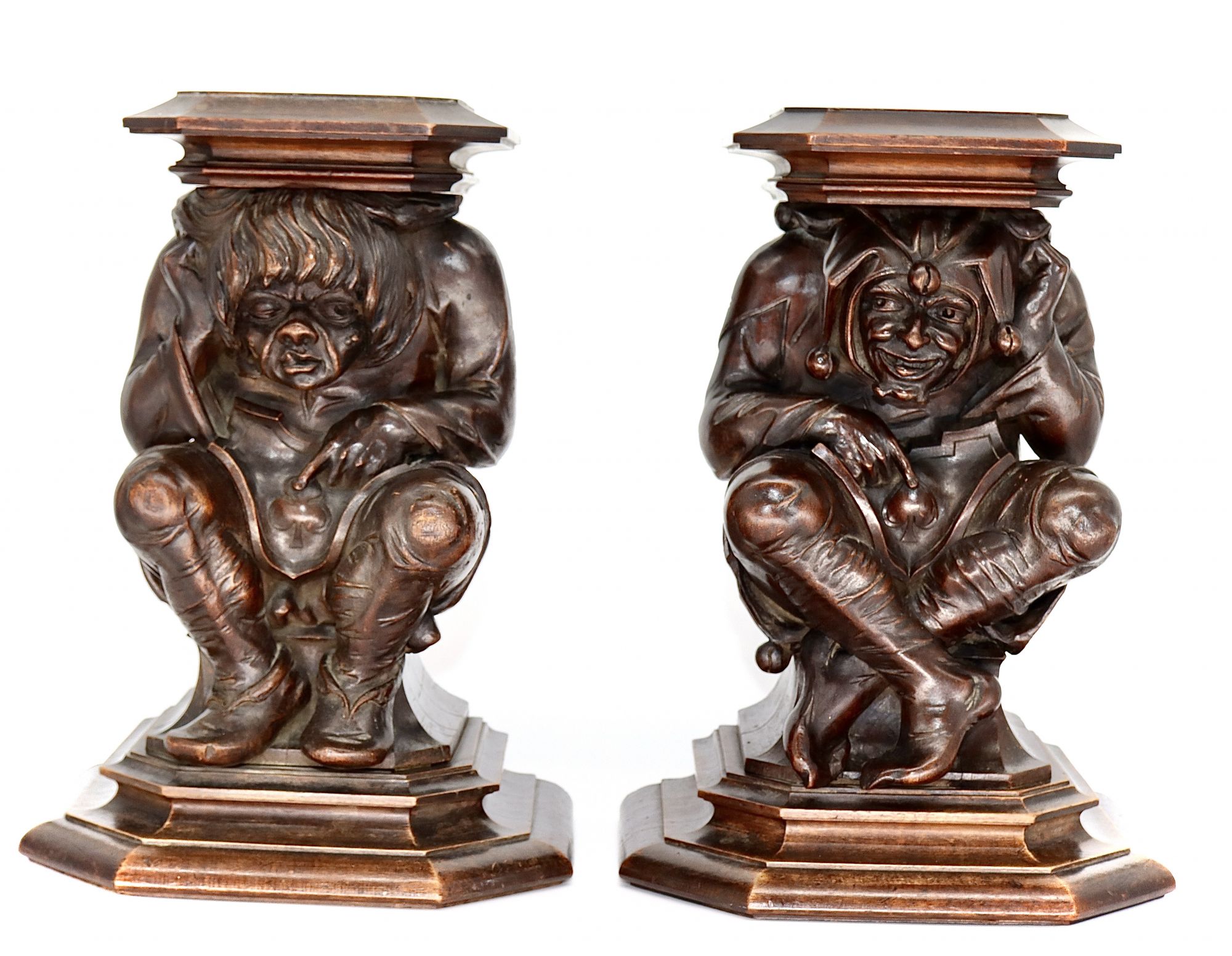This photo showcases two separate metallic statuettes, each functioning as either side tables or decorative pillars. Both pieces share a bronzed, reddish-burgundy hue. The statuette on the left depicts a deformed, goblin-like figure with long, curly hair and a tooth protruding from its mouth. Its facial expression appears dopey and glazed over. This figure, slumped with its head resting against the tabletop, has one hand on its knee and the other pointing towards a clover-shaped belly button. Additionally, it sports little booties. The statuette's top surface resembles a book lying flat on its back.

In contrast, the figure on the right exudes cheerfulness, akin to a court jester, and wears a distinctive jester's hat. This enigmatic character has a mischievous grin and cross-legged posture, with one hand pointing towards a spade-shaped symbol at its belly, and the other assisting in balancing the tabletop on its head. It also wears similar booties. Both figures, detailed with expressive features and unique props, provide a whimsical and intricate addition to the composition.